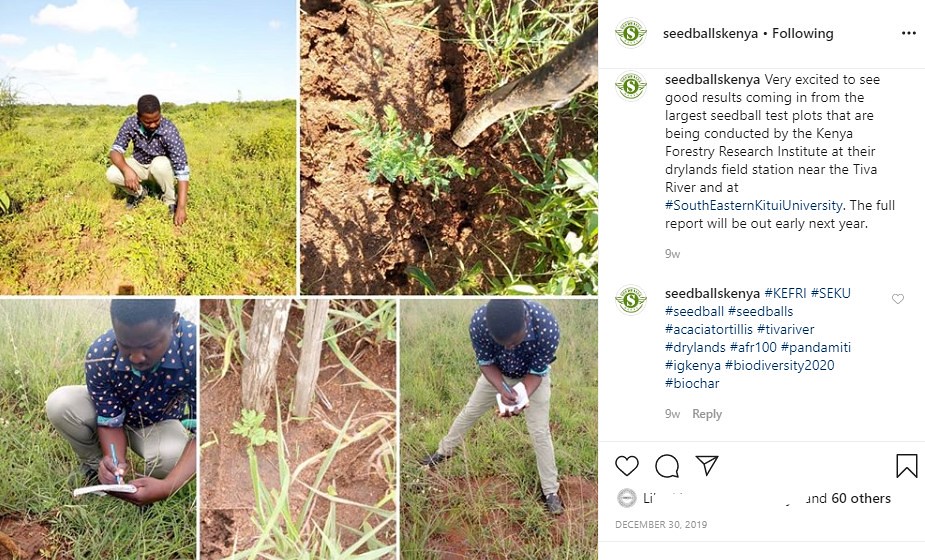The screenshot of an Instagram post by Seeds Ball Kenya displays a collage of five photographs on the left and text on the right. The text, posted on December 30, 2019, expresses excitement about the promising results from the largest seed ball test plots conducted by the Kenya Forestry Research Institute at their Drylands Field Station near the Tiwa River and at Southeastern Kitui University. The full report is anticipated early next year. The hashtags used include #KefriSekuSeedBalls, #AkakiaTortillus, #TiwaRiver, #Drylands, #AFR100, #PondaMiti, #IGKenya, #Biodiversity2020, and #Biochar.

The photographs, arranged in a collage style, feature a young African man, possibly a student or researcher, diligently studying a grass field. In the first image, he is bending down in a blue or dark navy shirt and beige pants, touching the grass. The second image provides a close-up of soil beside a tree trunk. The third image shows the same man bent over, taking notes in a journal. The fourth image displays grass in various growth stages, and the fifth portrays the man squatting to jot down notes. The visual arrangement consists of two square photos on top and three vertical photos underneath, forming a larger square. The text next to the images emphasizes the ongoing research and the positive developments in biodiversity efforts.